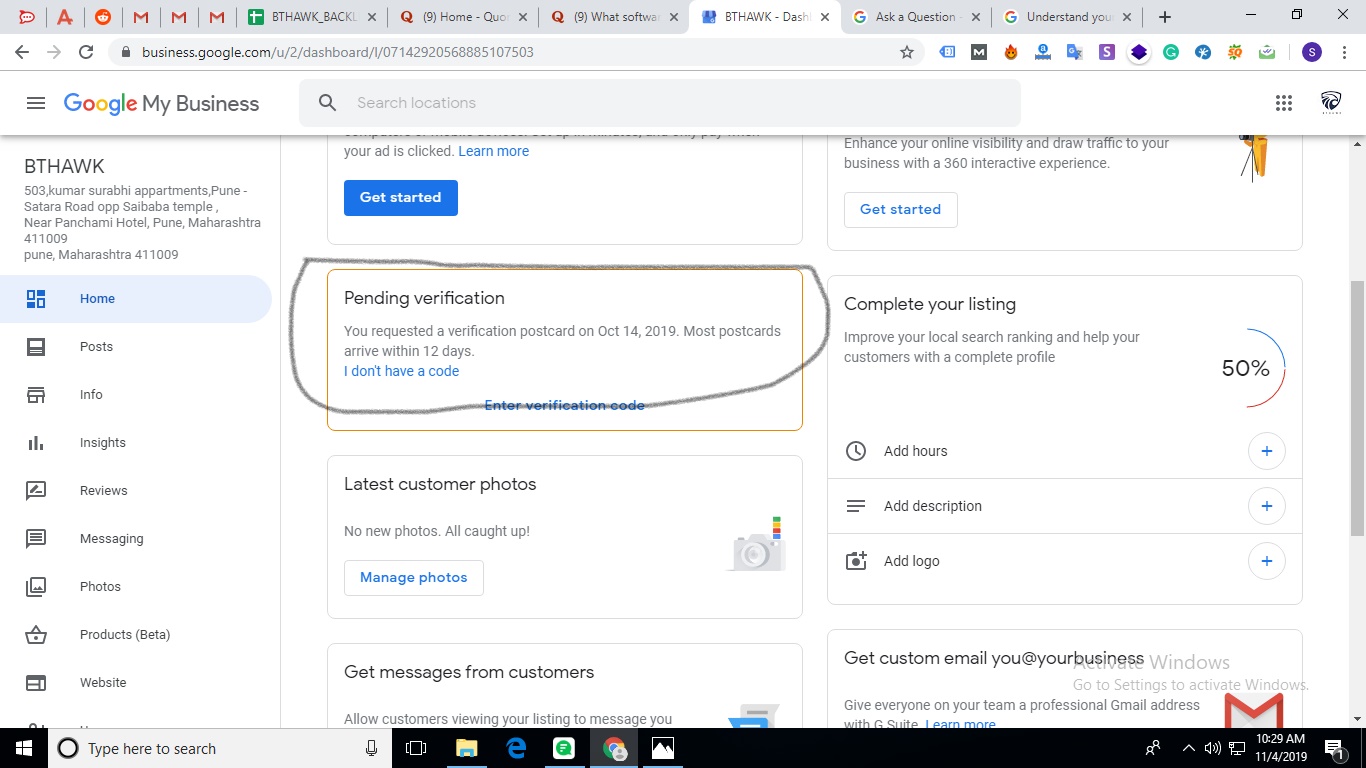Screenshot of a browser window displaying multiple open tabs, including two Quora tabs, one BT Hawk tab, and two Google tabs. The active tab is from BT Hawk and shows the URL "business.google.com/you/two/dashboard/one/[long number]". The page is titled "Google My Business" and features a search bar beneath the title. On the left side of the screen, there is a white-colored menu with the heading "BT Hawk". The main content area of the page is also white and contains a rectangle encircled in red labeled "pending verification". The text within the rectangle indicates that a verification postcard was requested on October 19, 2019, and mentions that most postcards typically arrive within 12 days, along with a note stating "I don't have a code".